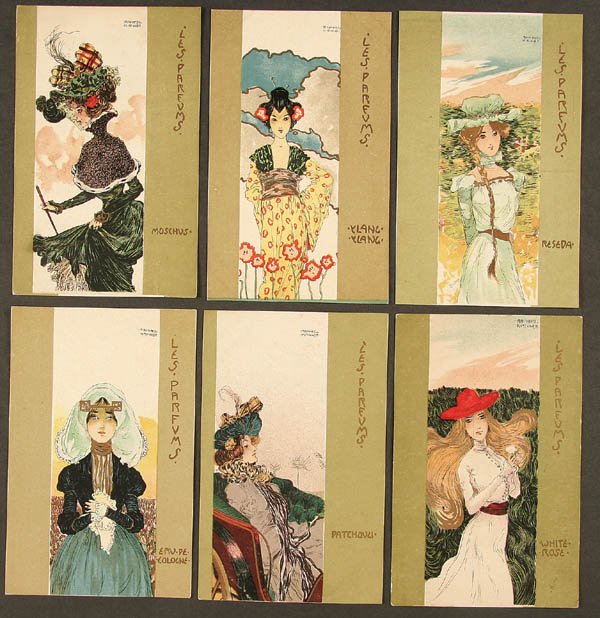The image depicts a set of six portrait cards arranged in two rows of three. Each card features a finely detailed illustration of a woman, bordered by thin, ornate gold strips on both sides. The right-sided gold strip contains intricate, darker yellow lettering, while small black letters, written in black ink, appear in the top right corner of each card. 

Starting from the top left, the first card shows a white woman in a green Victorian dress adorned with a brown scarf, holding a cigarette holder, and wearing a heavily decorated green hat. The second card portrays an Asian woman in a yellow kimono, complemented by a pink scarf and red flowers in her dark hair, styled with traditional pins. The third card, also on the top row, features a woman in an old-style light blue dress standing in a green field.

Moving to the bottom row, the fourth card displays a woman clad in a dark blue top with a matching fluffy skirt and a whitish-blue veil, looking straight ahead. The middle card on this row presents a seated woman in a gray coat with a green hat and a matching green scarf around her neck. Lastly, the bottom right card shows a woman with long blonde hair wearing a red cowboy hat, a white dress with a red belt, standing in a field.

All six cards share a uniform design with gold borders and thematic elements of historical, culturally rich attire, blending colors, and various settings that range from intricate backgrounds to simple fields.